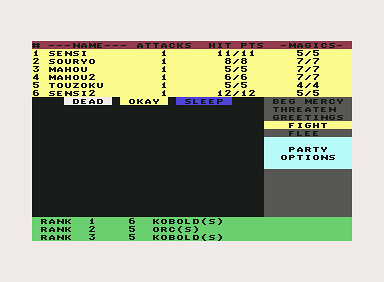The image is a screenshot from an old, party-based, turn-based RPG game, predominantly text-based. The on-screen display features various information boxes and rankings. The background is primarily a white or very light gray, with a red banner at the top listing headings like "Name," "Attacks," "Hit Points," and "Magics." Below this, a yellow line enumerates six party members: Sensei, Sarvo, Mahou, Mahou 2, Tozuku, and Sensei 2, each with corresponding statistics. To the right of these names are different states such as "Dead," "Okay," and "Sleep." At the bottom, a green-bordered area details player rankings with labels like "Rank 1," "Rank 2," "Rank 3," and enemy designations such as "kobold" and "orc." The screen also displays actionable options like "Fight," "Flee," "Threaten," and "Beg Mercy," with "Fight" currently highlighted, illustrating the party's menu choices. The image has a classic, vintage computer aesthetic, marked by an off-white, cream, or light gray border encasing the inner game display.